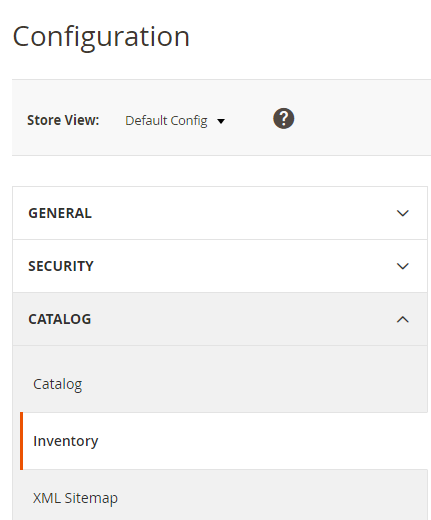A detailed depiction of a configuration window interface:

At the top left corner of the image, the word "Configuration" is displayed in a larger, thin, black font, with the letter 'C' capitalized and the entire text left-justified. This word stands out among the other elements on the screen due to its size.

The top bar of the window has a white background, contrasting with the gray bar directly beneath it. Positioned in the left-center of this gray bar, the text "Store View:" is rendered in smaller, bold, black font. Immediately following this text is a non-bolded phrase "Default Config," accompanied by a dropdown arrow indicating a selection option. To the right of this text, a black circle encloses a white question mark, serving as a help icon.

Below this gray bar, there is a spacing followed by a new section containing various categories listed vertically. These categories are:
1. General
2. Security
3. Catalog
4. Inventory

The "Catalog" category has an expandable dropdown menu, inside which the word "Catalog" appears again, indicating additional configurable options within this category.

This configuration window appears neatly organized, with distinct sections and consistent use of colors and fonts to differentiate the elements.